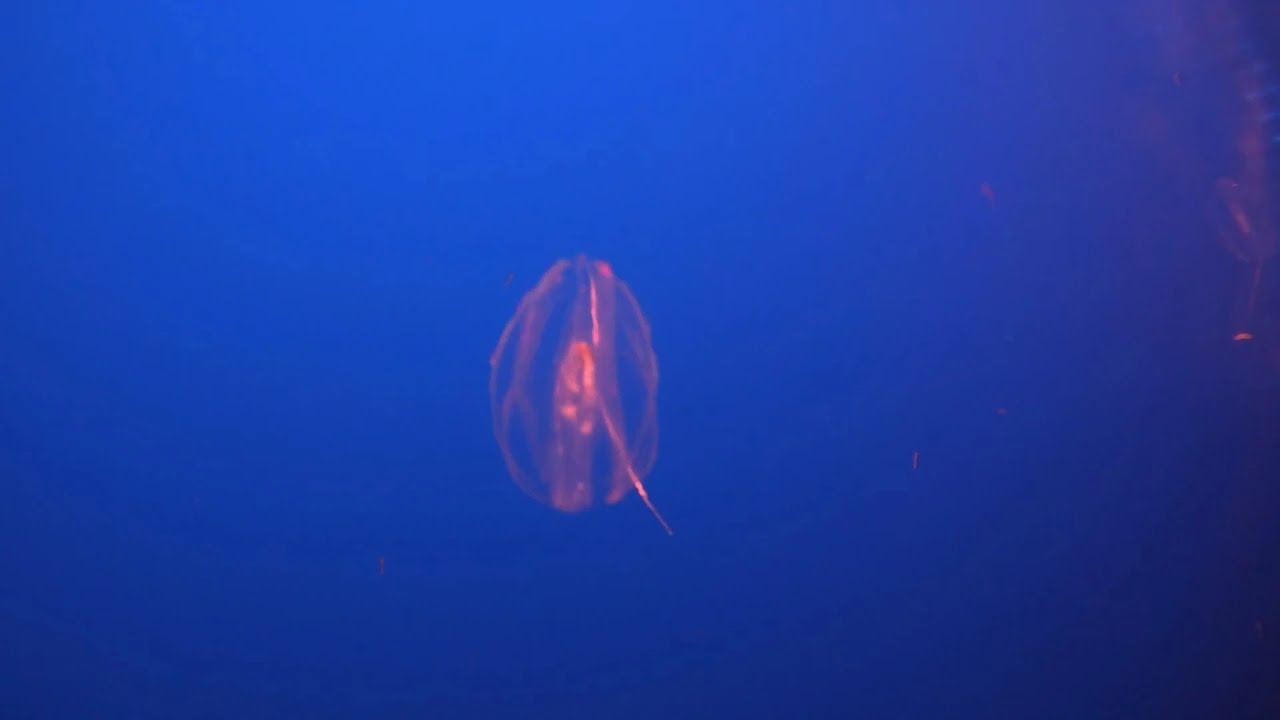The image presents a striking underwater scene set against a backdrop of deepening, rich royal blue that fades into black at the lower corners, with slight coral pink cloudiness at the top right edge. Dominating the center, slightly to the left, is an otherworldly figure resembling a jellyfish. This oblong, egg-shaped organism appears almost diaphanous, radiating alternating shades of coral, salmon pink, and red. The jellyfish's translucent body reveals the blue water behind it, while its inner portion glows with intricate, organ-like structures, enhancing its ethereal presence. The entire scene is solitary, with the vibrant blue darkness of the deep ocean highlighting the luminous, coral-hued jellyfish at its core.